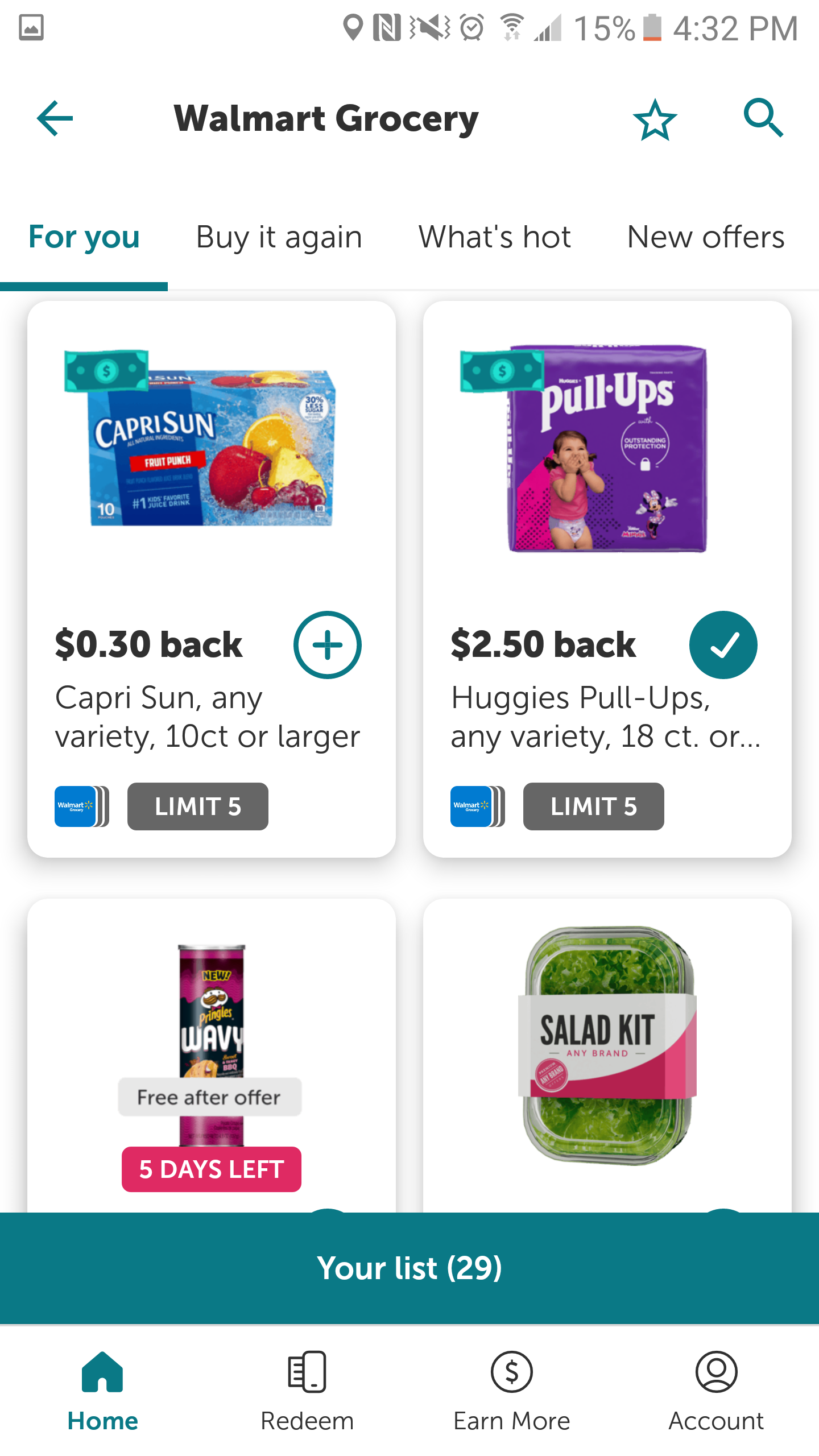This is a detailed screenshot of the Walmart Grocery app. At the top of the phone's display, the battery level is critically low at 15%, and the time is 4:32 p.m. There are multiple notifications visible in the phone's notification bar. 

Below the notification bar, the app interface prominently displays "Walmart Grocery" in the center of the screen. To the right of the title, there is a star icon and a magnifying glass icon for search. To the left, an arrow points to the left, indicating a back navigation option.

The app has several navigational tabs at the top: "For You," "Buy It Again," "What's Hot," and "New Offers." The "For You" tab is currently selected. Under this tab, four different items are displayed:

1. **Capri Sun**: A 10-count or larger box of Capri Sun with 30 cents cashback.
2. **Huggies Pull-Ups**: An 18-count or larger package of Huggies Pull-Ups with $2.50 cashback. A blue check mark indicates this item has been selected for purchase.
3. **Wavy Pringles**: Available for free after the offer, with five days remaining to claim the offer.
4. **Salad Kit**: An image of a salad kit is shown, though no specific offer details are provided.

Beneath these items, there is a "Your List" button indicating that the user has 29 items saved on their list. At the bottom of the app interface, a toolbar includes several options: "Home," "Redeem," "More," and "Account."